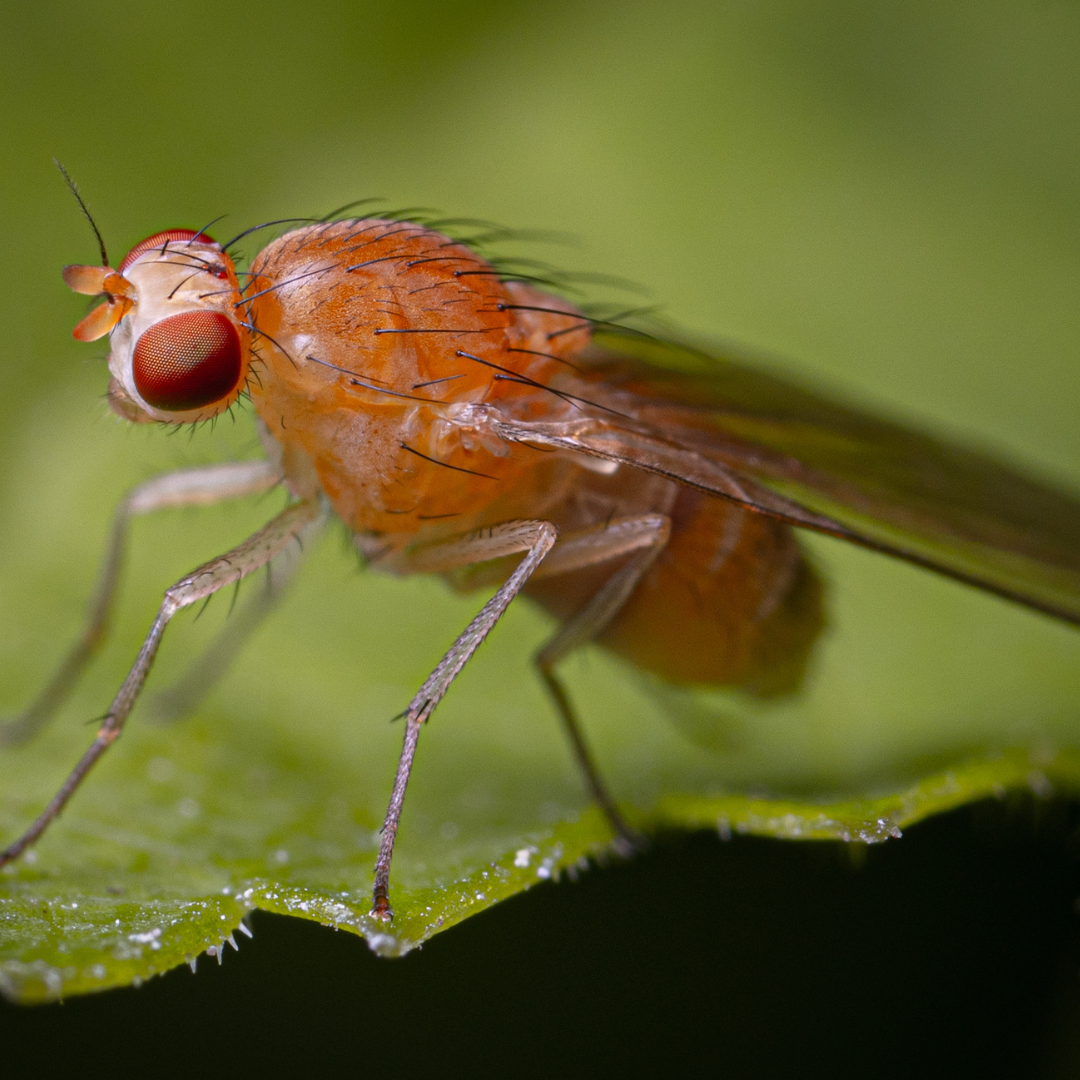The photograph is a detailed close-up of a small, fly-like insect with an orange-beige body, standing on a blurred green leaf. The insect's side view showcases its semi-transparent, silver-colored legs and brownish, translucent wings tucked neatly along its back. The insect has large, striking red eyes and a head that faces the left side of the image. Its body and head are covered in tiny black hairs, adding to its unique appearance. The leaf it rests on is green, but blurred, with a dark area at the bottom of the image providing contrast. The photograph captures the insect's intricate details, making it an impressive and distinctive shot.